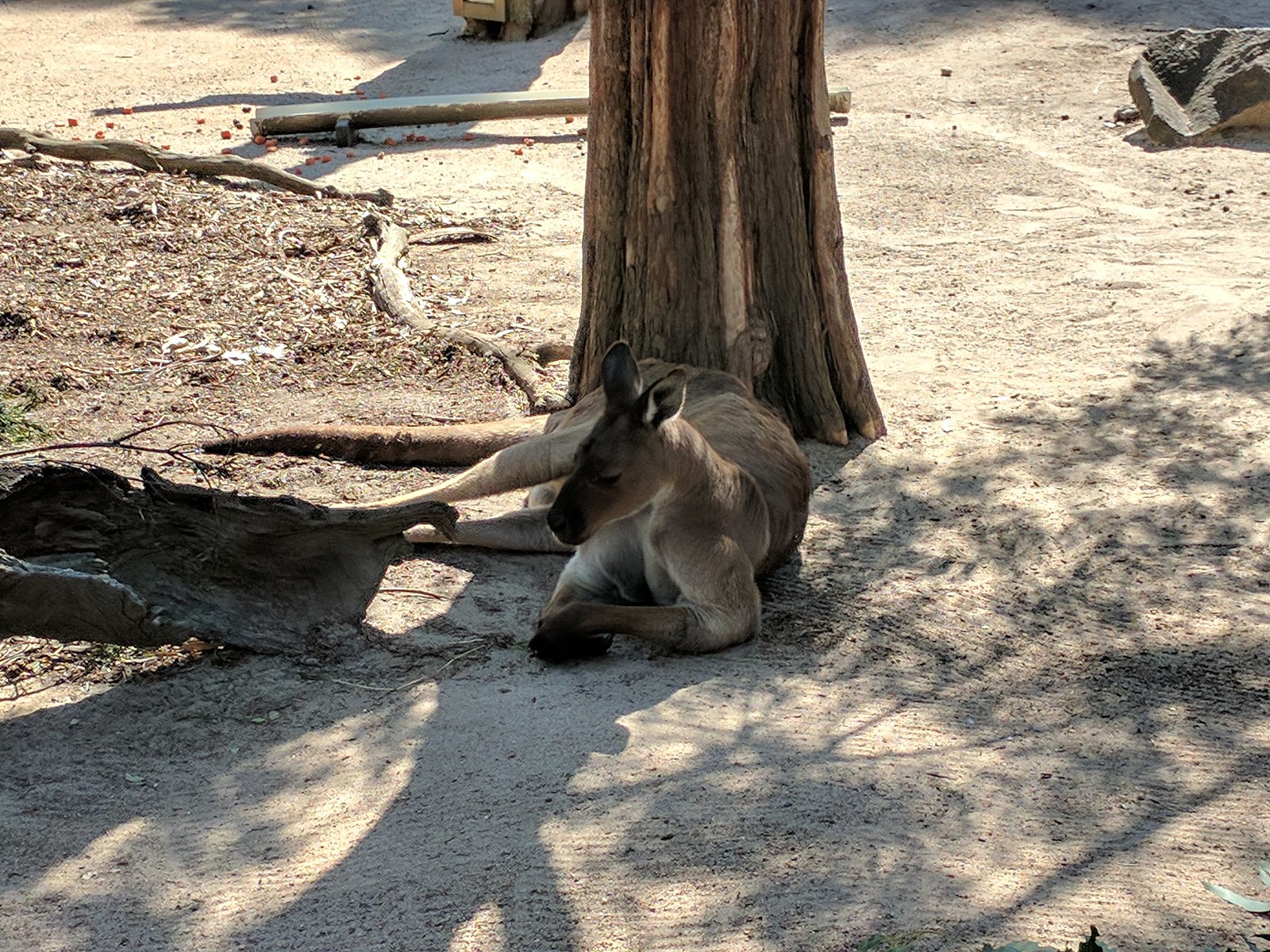The image, taken outdoors during the daytime, depicts a lounging kangaroo in a shaded area. The scene is rectangular, wider than it is tall, focusing on light, sandy dirt ground marked with rake patterns, particularly noticeable at the bottom. In the mid-center lies a brown kangaroo, its body facing to the right with outstretched legs and tail to the left. The kangaroo’s underbelly is a lighter cream color contrasting its light brown coat. Its paws, with tips dark brown to almost black, stretch out front, and its similarly colored darker muzzle is tipped downwards, facing left. The creature appears relaxed, possibly sleeping with closed eyes.

To the left of the kangaroo is the shell of a dead log, primarily its bark, and behind it stands the trunk of a brown tree extending vertically. Visible roots meander at the topsoil level. The background features patches of dead leaves to the left and a large stone rock in the upper right corner, bathed in sunlight, unlike the shaded area where the kangaroo resides. An open space with sunlight and additional tree roots occupy the backdrop, suggesting a tranquil and possibly contained environment like a zoo or wildlife refuge, inferred from the appearance of structures, such as a trough-like half barrel on little supports.